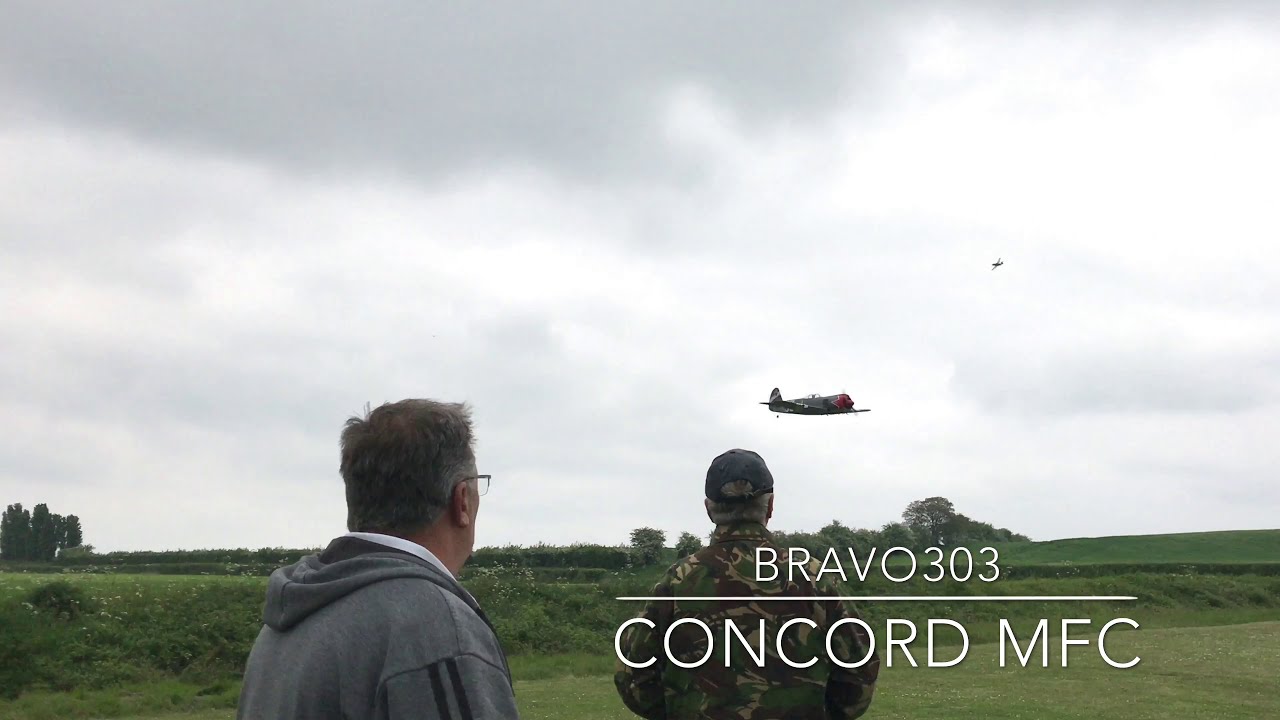In this detailed outdoor scene, two men stand on a flat, green landscape, watching an airplane fly low in the sky. The sky above them is blanketed with light gray and white clouds. Greenery covers the ground, with a mix of lighter grass in the foreground and darker shades in the middle and background, along with a few scattered trees. The man on the left wears a gray sweatshirt with black stripes on the arms, has thin graying hair, and glasses. The man on the right is dressed in a long-sleeve camouflage jacket and a black hat. Both men have graying hair and are staring intently at the airplane. The aircraft, resembling an old World War II fighter plane, features a silver body and a red front near the propeller. Additional features in the sky might include another small plane or birds. Text at the bottom right of the image reads "Bravo 303, Concord MFC" in white font.